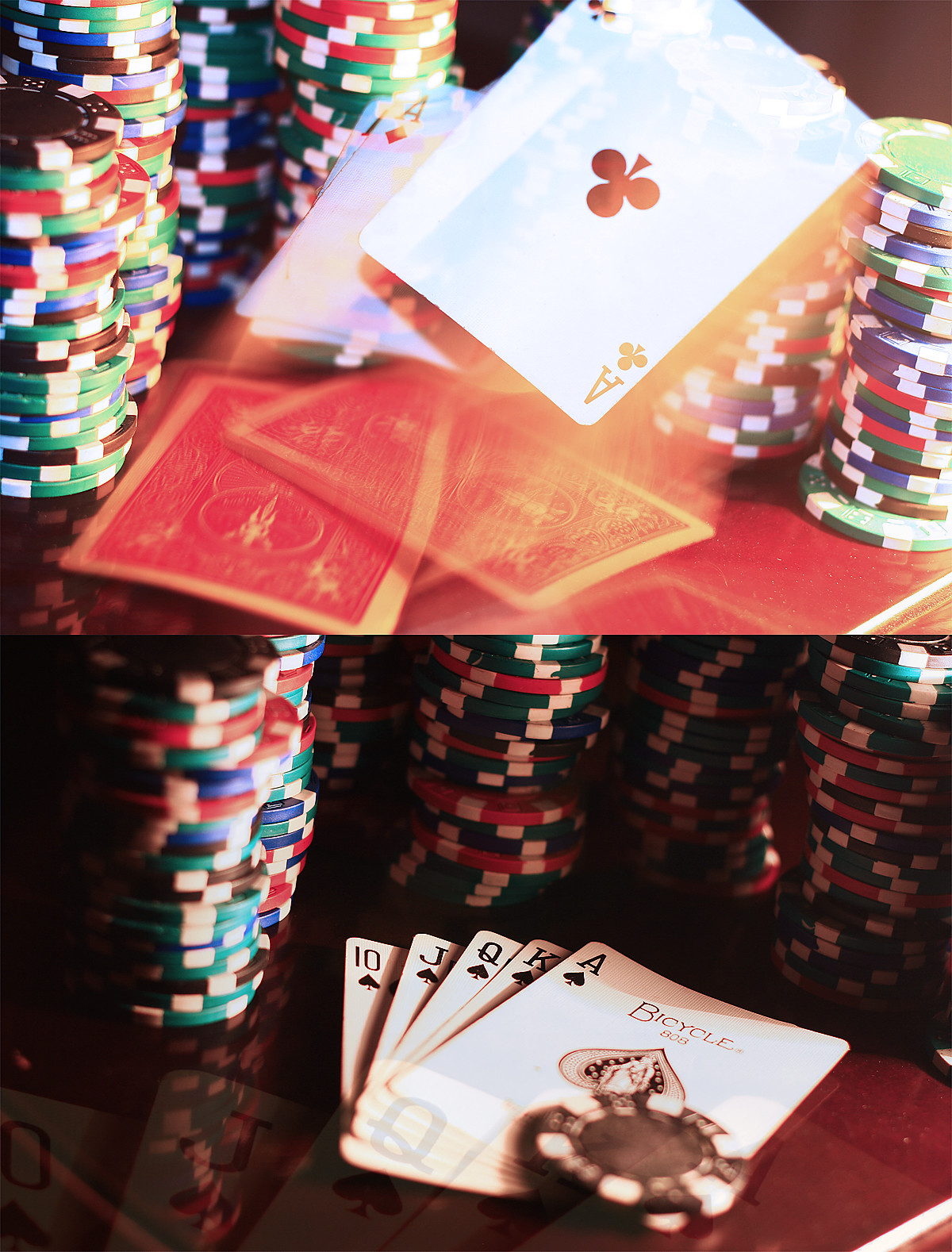**Top Photograph**: The image prominently displays an assortment of poker chips meticulously organized into stacks on a vibrant red table. The chips are primarily green, red, blue, and black, each adorned with white accents around their perimeters. Positioned in the midst of these chips are two playing cards, with the Ace of Clubs displaying its distinct black club symbol at the top, partially covering the Ace of Diamonds beneath it. One card appears to be sliding onto the other, enhancing the dynamic visual effect.

**Bottom Photograph**: This second image, captured on the same red table under slightly dimmer lighting, offers a different perspective of the poker chips and cards. The stacks of chips are visible, but the focus shifts to a straight flush in Spades, perfectly arranged from top to bottom. A black poker chip rests atop the Ace of Spades, leading the sequence of King, Queen, Jack, and Ten of Spades, presenting an impressive poker hand. The darker ambiance and subtle angle contrast with the first image, enriching the overall depiction of a classic poker game setup.